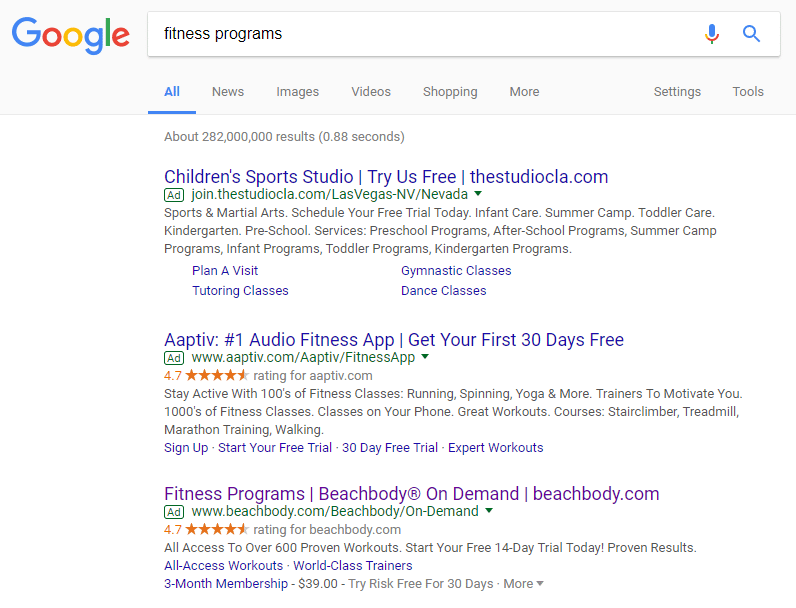This is a detailed screenshot of a Google search results page. At the top left, the familiar Google logo is displayed with a blue "G," a red "O," a yellow "O," a blue "G," a green "L," and a red "E." Below the logo lies the search bar, which is white with a light gray border, containing the query "fitness programs." 

Directly underneath the search bar are several tabs: "All" (which is highlighted), "News," "Images," "Videos," "Shopping," "More," "Settings," and "Tools." Below these tabs, the page indicates that approximately 282 million results were found in 0.88 seconds. 

The first search result is a paid advertisement for "Children's Sports Studio." The result is from the website join.thestudiocla.com/las-vegas-nevada and features a green-outlined box labeled "Ad." There is a dropdown in the same green hue. The description mentions offerings such as sports and martial arts, infant care, after-school programs, and infant programs. It highlights four categories: "Plan a Visit," "Tutoring Classes," "Gymnastic Classes," and "Dance Classes."

The second search result is an ad for "APTIB" – touted as the number one audio fitness app. The user can get their first 30 days free. The website address, displayed in a green font, is aptib.com, and it is accompanied by a green "Ad" box. This result boasts a 4.7-star rating and offers various services such as spinning, yoga, great workouts, stair climber, and more. At the bottom, there's an option to sign up for a free trial.

The third search result is for "Beachbody On-Demand" from beachbody.com, which is displayed in purple, signifying a visited link. This result too has a green "Ad" box and a 4.7-star rating. It promotes access to over 600 proven workouts with a three-month membership for $39.